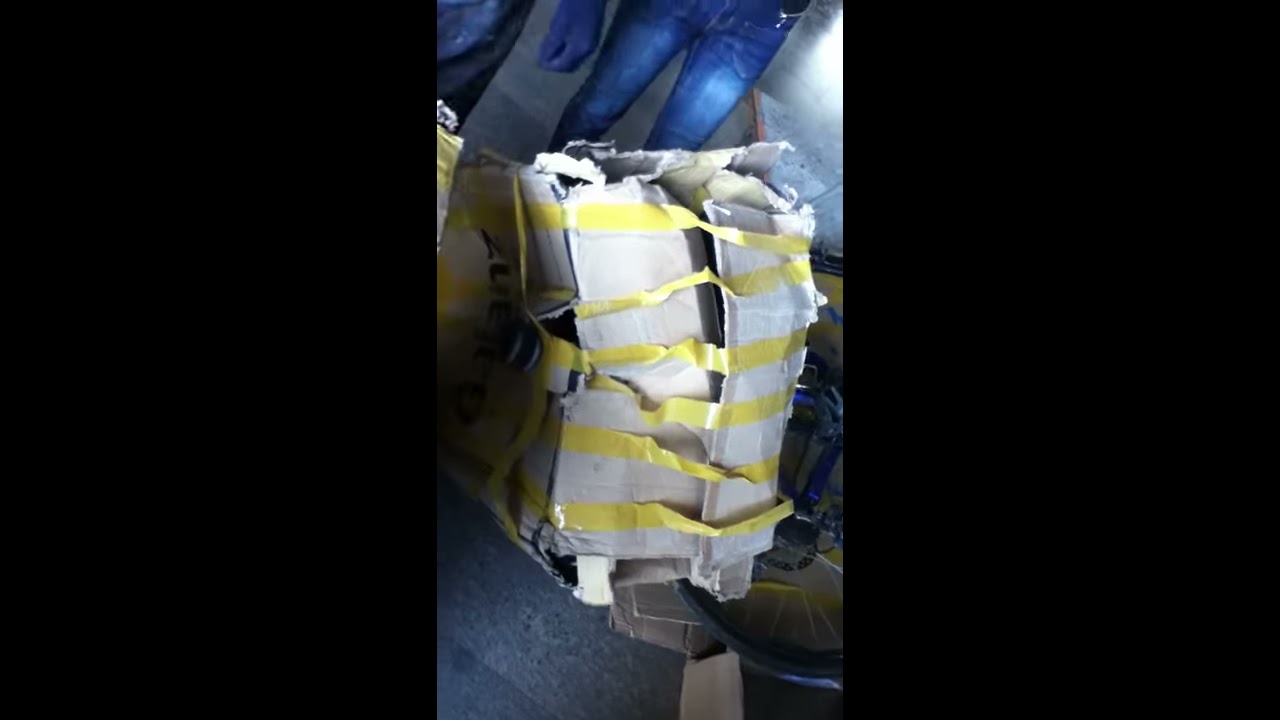The photograph depicts a heavily damaged and crushed white box situated in the center. The box is secured with six strips of yellow tape, spaced uniformly from top to bottom, holding the box together amidst visible tearing and creasing. In the upper part of the image, a person wearing blue jeans and a blue glove is slightly visible, suggesting a possible action or scene involving human activity. The background reveals a somewhat industrial or storage-like setting, likely a warehouse or garage, indicated by the concrete floor. The right and left edges of the image are enveloped in darkness, with only a subtle light illuminating the scene from the right, casting some parts of the background in lighter hues. The box has patches of gray near the taped areas, adding to the impression of wear and tear. No text or words are present in the image.